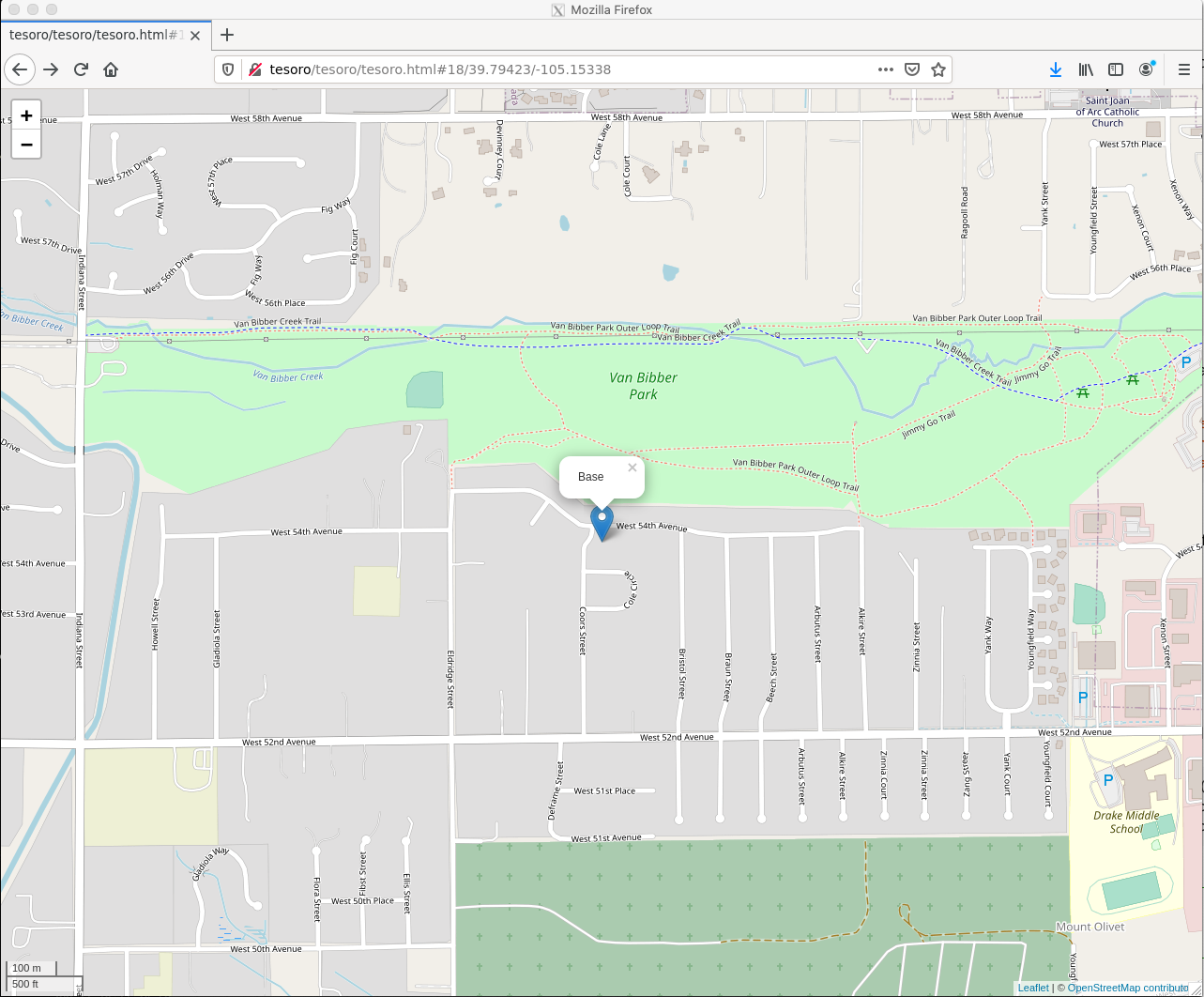This image is a snapshot of a map from the Tesoro website. At the center of the map is a blue pen mark with an accompanying speech bubble labeled "BASE," indicating a specific point of interest. This point is located on a street directly across from Van Biber Park. The name of the street is illegible due to the small font size; however, it is depicted as running horizontally, suggesting an east-west orientation. Around this horizontally running street, several other streets branch off in a north-south direction. In the bottom right corner of the map, Drake Middle School is visible, showing that the marked street is within walking distance of the school while being closer to Van Biber Park. Additionally, a major road can be seen situated to the north of the park, highlighting its connectivity to broader routes.